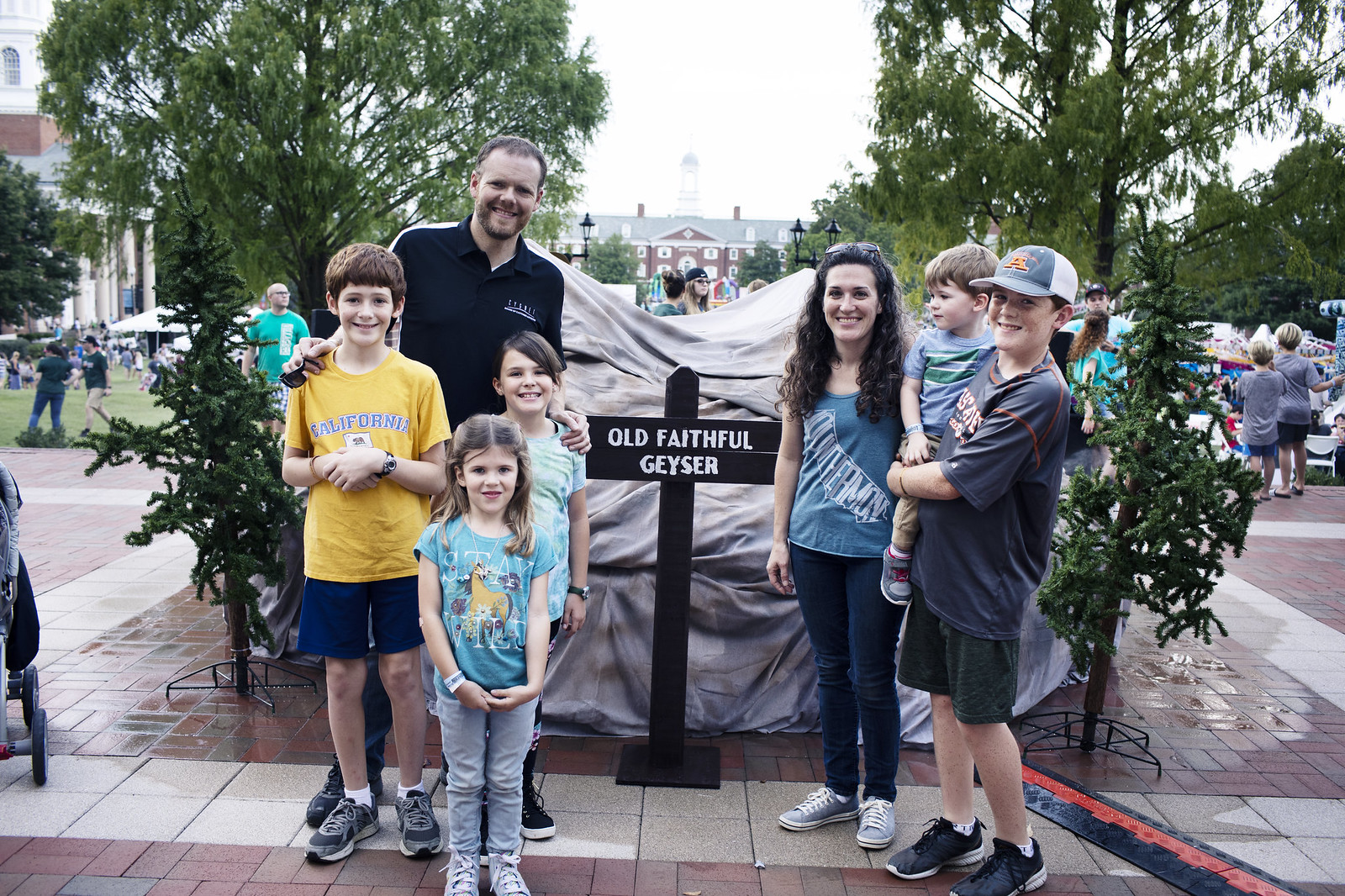In this family photo, taken on a brick patio in what appears to be a bustling college quad or park area, a mother, father, and their five children are all smiling at the camera. To the right of the photo stands the mother with long curly hair, wearing a blue shirt and jeans. Beside her is their approximately 12-year-old son in a blue T-shirt, green shorts, and a ball cap, holding their youngest child, a toddler in a blue shirt. On the left side, the father, donned in a dark blue shirt, stands slightly in the background, with an 8 or 9-year-old boy in a yellow T-shirt standing in front of him. Next to this boy is a 7-year-old girl, and in front of the siblings is another young girl, possibly 6, wearing jeans and a blue shirt.

Between the parents stands a prominent black sign reading "Old Faithful Geyser." However, the scene is evidently not the actual geyser; instead, it features a large, gray-sheet-covered object behind the family, flanked by artificial trees on either side, likely a replica or monument. Surrounding them are historic buildings that could include structures akin to Independence Hall. Various college buildings envelop the background, with people milling about and some canopies suggesting a possible fair or market event. There's also a stroller nearby, indicating the toddler might have just been taken out for this picture. The sky looks cloudy, hinting at recent rain.